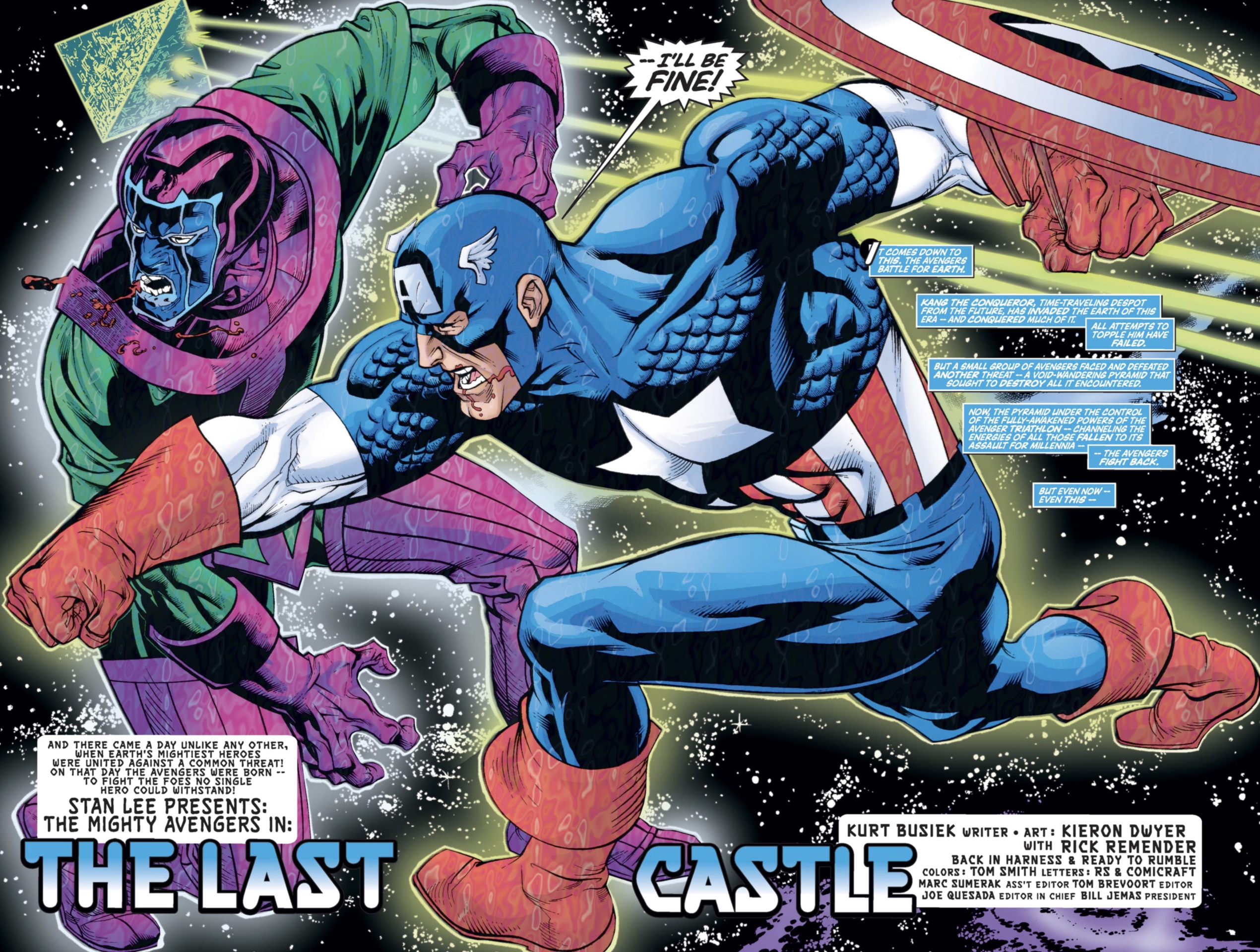The image is an advertisement for a Marvel comic book titled "The Last Castle," presented by Stan Lee as part of "The Mighty Avengers" series. The central focus is on Captain America, depicted in striking red, white, and blue attire. He is caught mid-action, lunging forward from a side angle, with his right arm extended in a powerful punch toward an off-screen foe, while his left foot steps forward and his shield is strapped to his left arm. To his left, a green and purple villain appears in the background, seemingly the target of his attack. The setting is space-like with a black background and white stars. Written text includes "I'll be fine" as a speech bubble, and a detailed caption at the bottom which mentions "The Last Castle" and credits writers Kurt Busiek, Kieron Dyer, and Rick Remender. The vivid, dynamic artwork captures the intense energy of the scene, emphasizing the heroic action of Captain America against his adversary.